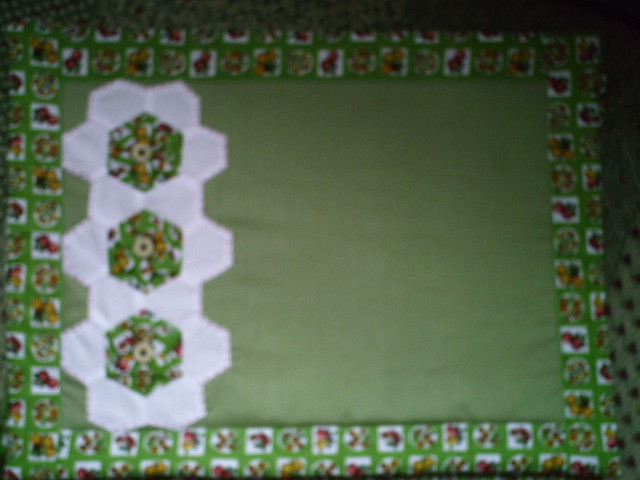The image is a horizontally aligned, blurry photograph capturing what appears to be a quilt, possibly a fabric placemat or pillowcase. The outer border is thick and decorated with colorful squares featuring various hues such as pink, brown, red, purple, and yellow, all set against a white background. Within the border, the central fabric is a solid, muted green. Catching the eye on the left side of this green expanse are three large, interconnected white flower shapes with hexagonal interiors. Each of these hexagonal centers repeats the colorful patterns found in the quilt's border, forming a harmonious design.